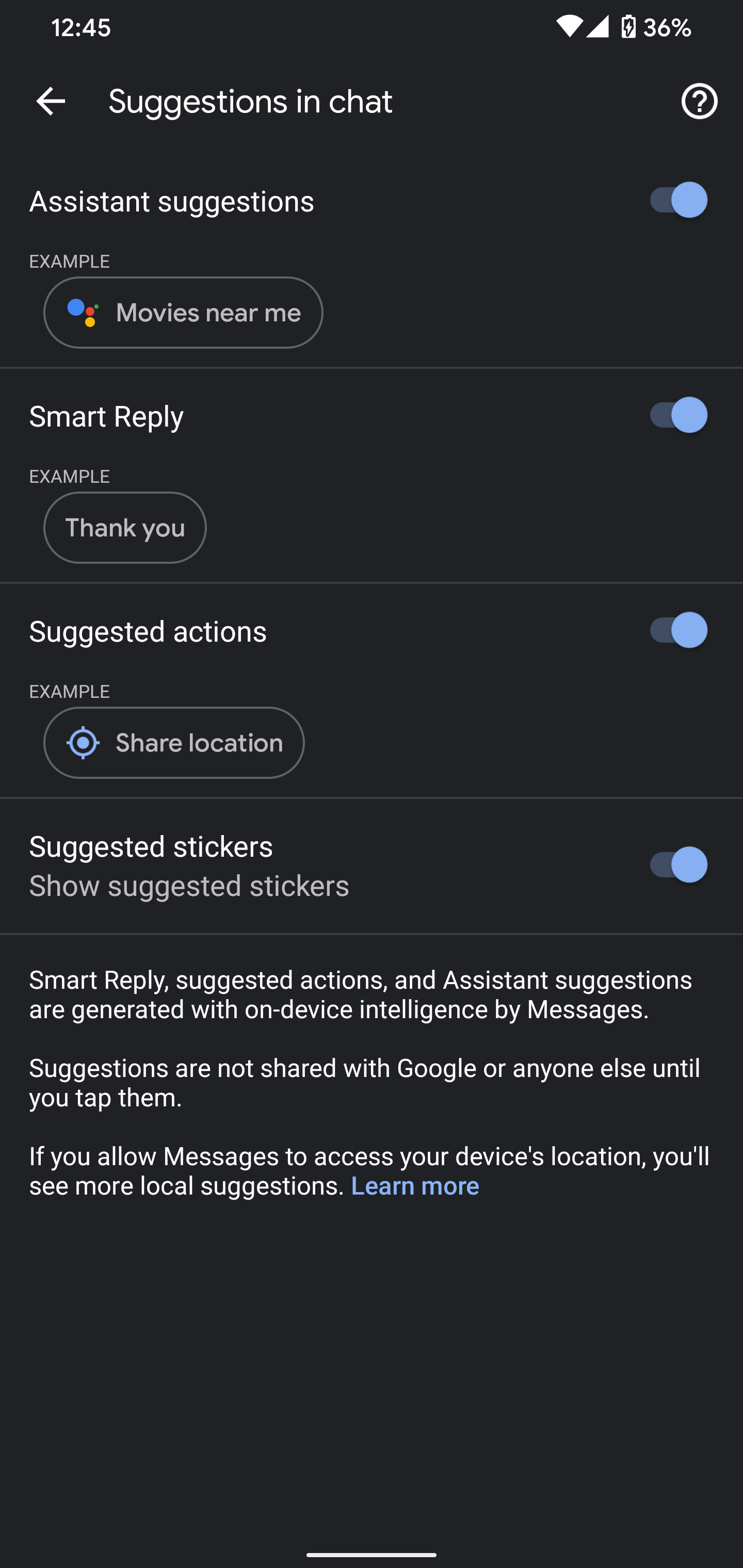This image appears to be a screenshot taken from a smartphone with a dark-themed interface. The background is predominantly black or dark gray, while the text is white for high contrast. 

In the top left corner, the time is displayed as 12:45, with the right side of the status bar showing several icons: a Wi-Fi indicator, a cellular signal indicator, and a battery icon indicating the battery is charging and currently at 36%.

The main content of the screen displays as follows:
- A back arrow, which likely navigates back to the previous screen.
- The title "Suggestions in Chat" is prominent, with a circle containing a question mark next to it, presumably for accessing information or help.
- Below it, the section "Assistant Suggestions" has a blue toggle switch that is turned on.
- An example suggestion labeled "Example: Movies Near Me" is shown below the assistant suggestions.
- The next section, "Smart Reply," also features a toggle switch in the on position and gives an example suggestion: "Thank You."
- Following that, "Suggested Actions" has its toggle switch turned on and includes an example with a location icon and the text "Share Location."
- "Suggested Stickers" also appears as a section with its toggle activated, and an option to "Show Suggested Stickers" is underneath.

At the bottom of the screen, there is an informative message in white text:
"Smart Reply, Suggested Actions, and Assistant Suggestions are generated with on-device intelligence by Messages. Suggestions are not shared with Google or anyone else until you tap them. If you allow Messages to access your device's location, you'll see more local suggestions."

The text "Learn More" is in blue, indicating it is a clickable link for further information. 

Finally, at the very bottom, there is a white line, likely a gesture indicator for accessing the device's navigation menu or app drawer.